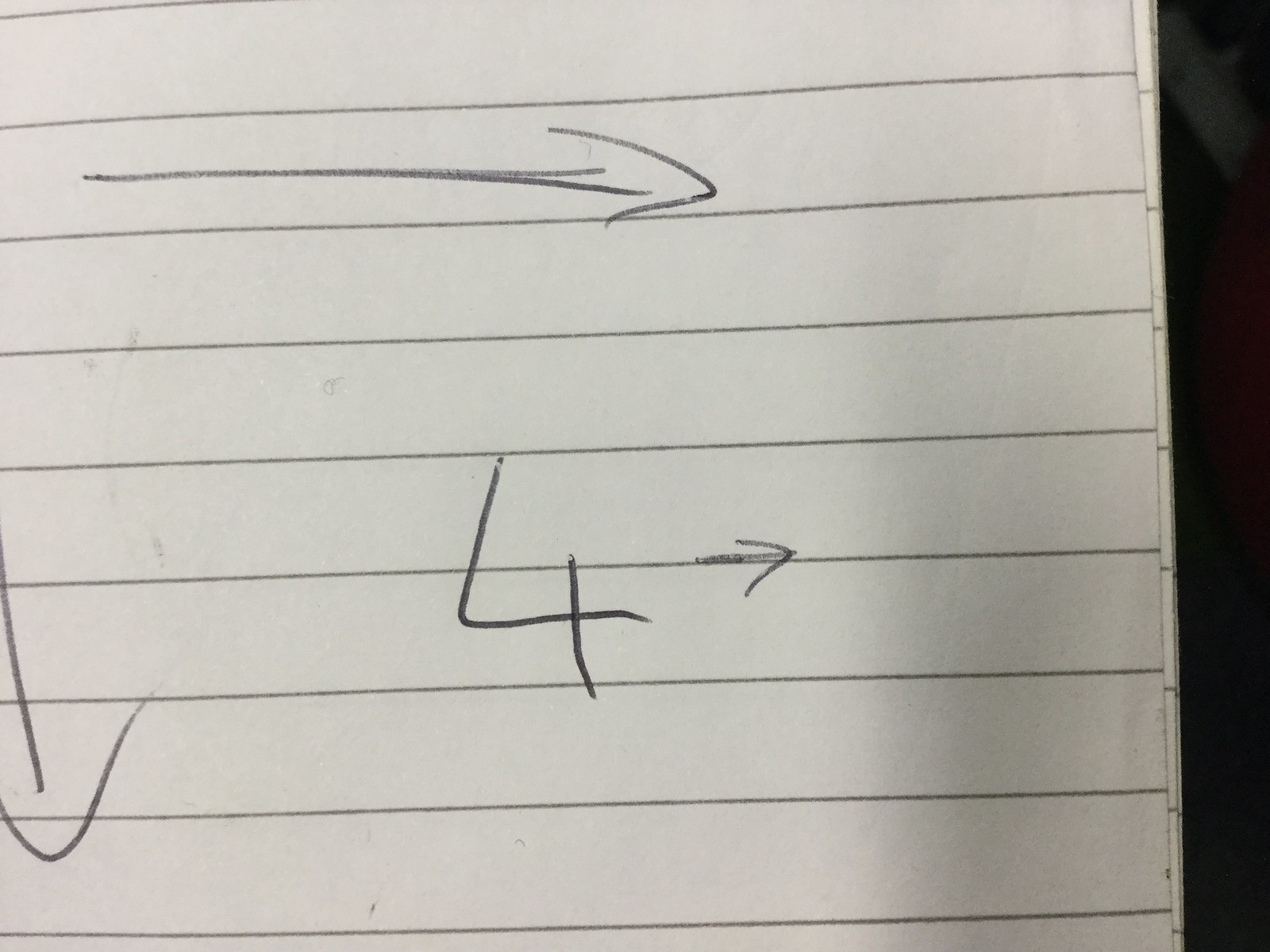A highly detailed close-up image captures a section of lined paper, showcasing eight horizontal blue lines and a partial ninth line at the bottom edge. The second line from the top features an arrow pointing to the right side of the photograph, indicating a direction towards the left side of the page. Below this, on the third line, there's another arrow, this one pointing downward on the left-hand margin. In the center of the paper, the number "4" has been written, alongside a small arrow also pointing to the right. Towards the far right edge of the paper, a dark, vertical line is visible, marking the boundary where the current sheet overlaps with another page or background object, the details of which remain indistinct due to the shadow. The paper itself appears slightly dirty, adding a textured, worn look to the overall image.